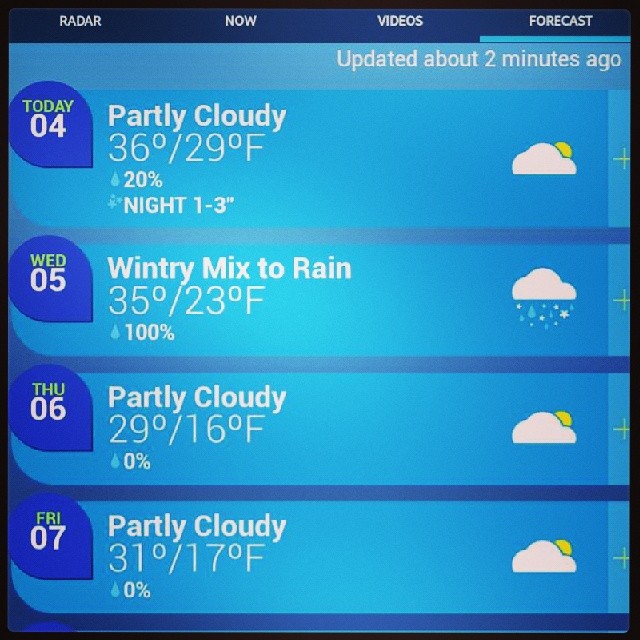The image is a screenshot of a weather app featuring a detailed forecast. The top of the screen includes a dark blue menu bar with tabs labeled "Radar," "Now," "Videos," and "Forecast" in red ink. Below that, a thin light blue line separates the menu from the main content, which has a blue background. At the top right of the main content area, it says "Updated about two minutes ago." The forecast is organized in rectangular strips, each representing a day. The days listed are: 

- **Today (04):** Partly cloudy, 36°F high, 29°F low, 20% chance of rain, with nighttime snow accumulation of 1-3 inches. 
- **Wednesday (05):** Wintry mix transitioning to rain, 35°F high, 23°F low, 100% chance of rain. 
- **Thursday (06):** Partly cloudy, 29°F high, 16°F low, 0% chance of rain.
- **Friday (07):** Partly cloudy, 31°F high, 17°F low, 0% chance of rain.

The left side of each strip displays the day and its date, while the right side shows corresponding weather icons: a sun peeking from behind a cloud for partly cloudy days, a combination of snowflake and raindrop for wintry mix, and sun above clouds for later forecasts.